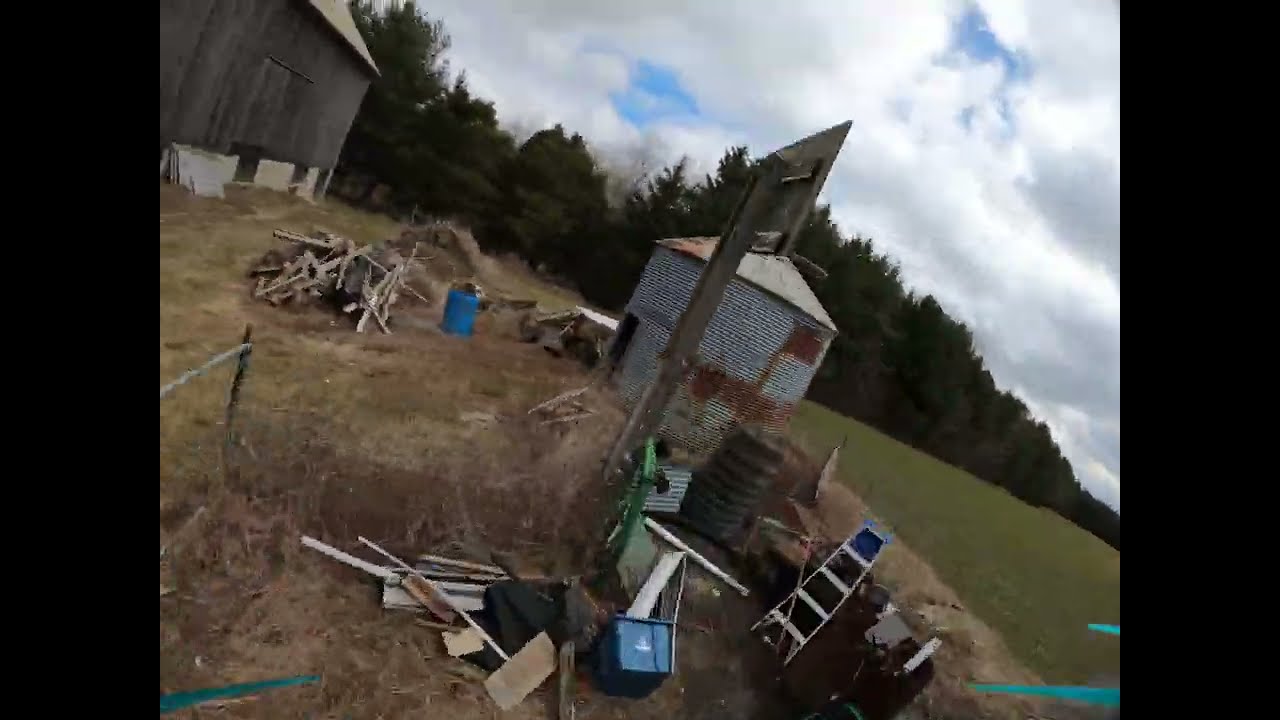The image depicts a cluttered farmyard scene, tilted slightly to the right. Dominating the top left corner is part of a brown farmhouse with a triangular roof, partially visible and with no windows. In front of the farmhouse lies a pile of wood logs, some hay, and a bright blue circular container. Near the center stands an old, rusted cylindrical silo with a dome-shaped top. The ground throughout the scene is covered in dry grass, twigs, and dirt, indicative of neglect. Scattered around are various pieces of lumber, debris, and tools including a ladder and a blue barrel. An old basketball hoop is somewhat visible among the chaos. In the distance, the scene is framed by a dense line of fluffy, pine-like trees stretching along the horizon under a mostly cloudy sky with patches of blue. The overall atmosphere suggests a remote farm or ranch far from urban areas.